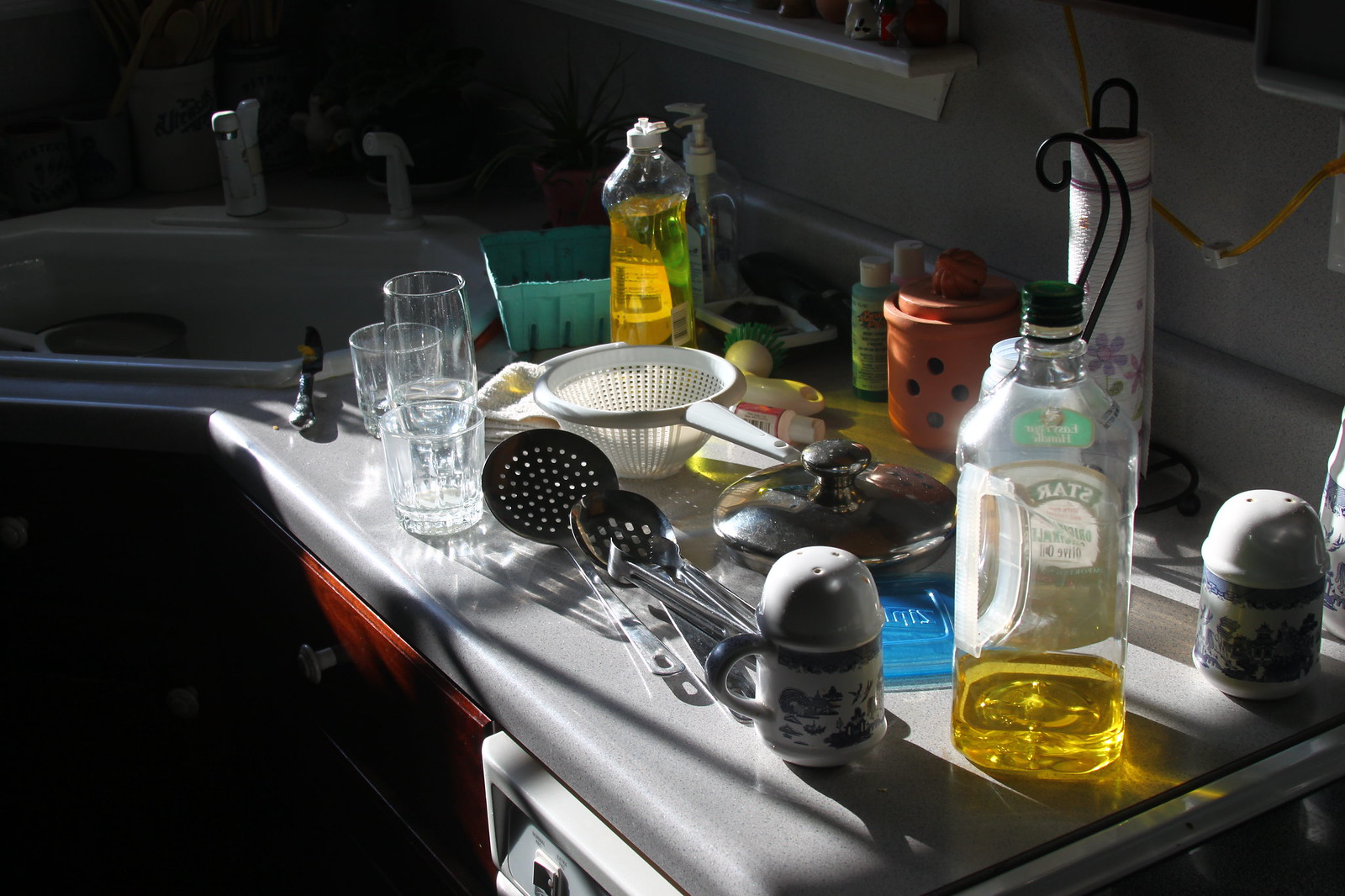The image depicts a cluttered light gray countertop situated between a sink and a cooktop, with a dishwasher nestled underneath a portion of it. The countertop hosts an array of items in disarray. There is a dish soap bottle, a green cardboard quart-sized fruit carton, and an assortment of clear drinking glasses varying in structure and height. A towel, a metal strainer, and a cooking pan adorned with its lid are also visible.

Additionally, a paper towel holder stands amidst the chaos, accompanied by a salt and pepper shaker duo and what appears to be a jug of oil or vinegar. A pair of tongs, two long-handled utensils with strainer ends, and the lid of a Ziploc container are scattered on the surface.

Among the clutter lies another soap dispenser, a hand cream tube, and yet another towel. Highlighting the scene, the lower cabinets beneath the counter and sink boast a vibrant red hue. Above, a pendant light hangs down, illuminating the countertop's eclectic assembly.